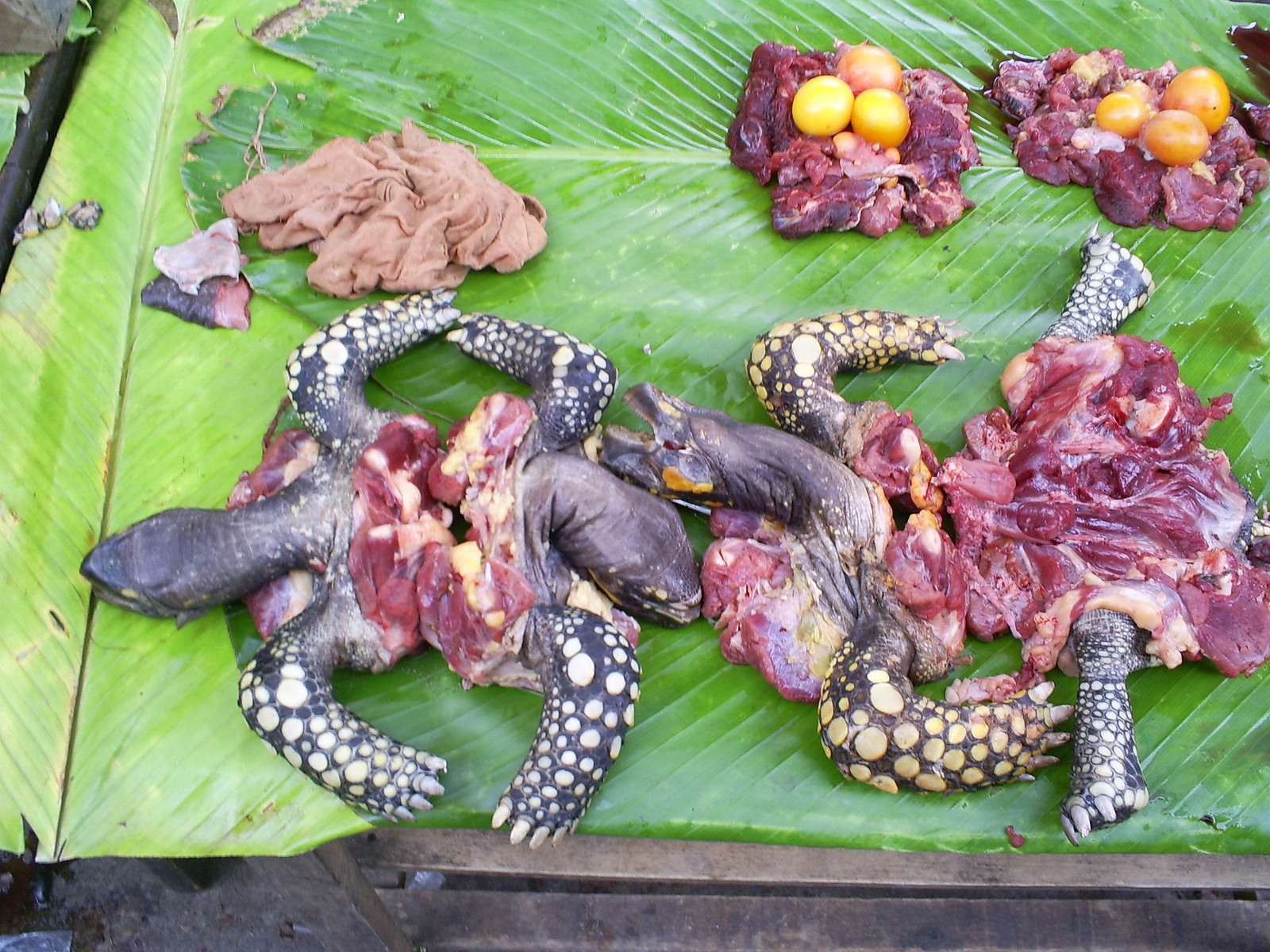The image depicts a disheartening and disturbing scene of animal cruelty. In the foreground, two disemboweled turtle bodies lie on a bed of large green leaves, possibly banana or palm leaves. Their shells have been removed, exposing raw red meat, and they appear to have been prepared for sale as food. In the background, two piles of meat are visible, each topped with what seems to be eggs, possibly turtle eggs, alongside some vegetables such as tomatoes. The unsettling and revolting nature of the image is palpable, especially for animal lovers, as it showcases the turtles in a brutalized state, highlighting an act of butchery likely intended for culinary purposes.